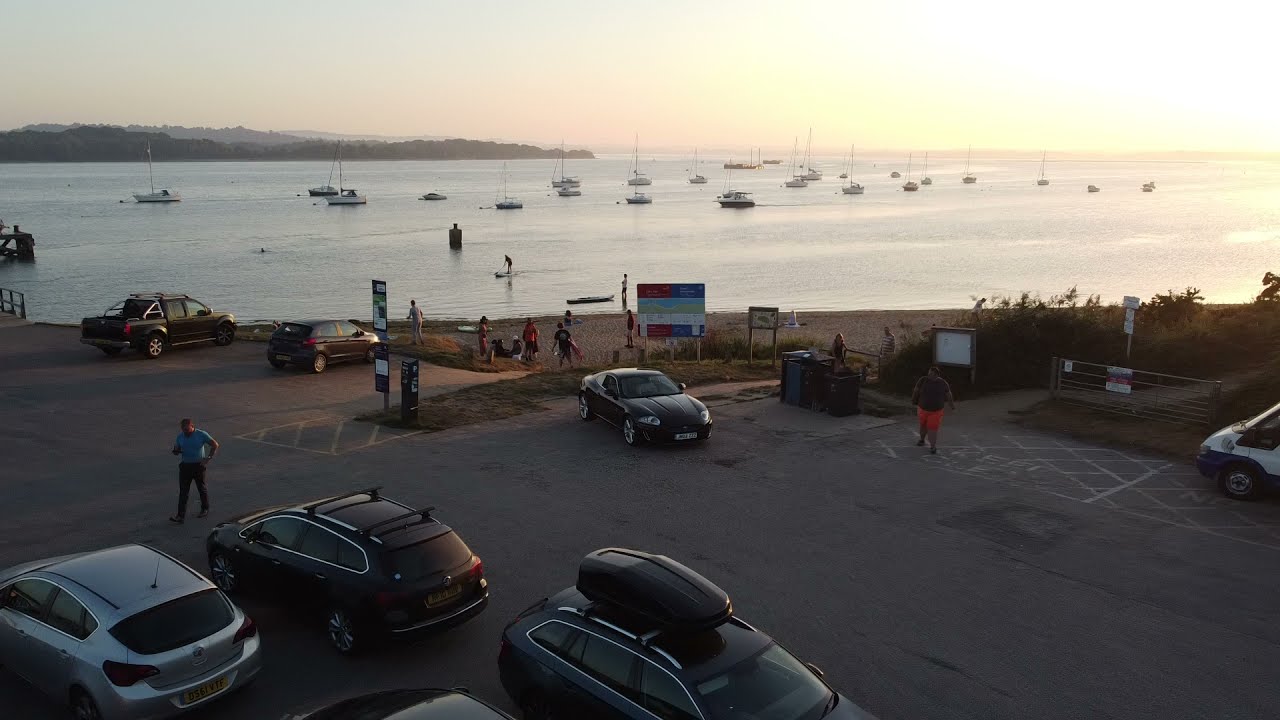The image captures an aerial view of a beachside parking lot during sunset. Four main vehicles are visible, including a dark-colored SUV with an egg-shaped object on the roof, a silver hatchback with an orange rectangular license plate, another SUV, and a sports car. The sun is setting on the far right of the image, casting a warm gradient of orange and pink hues across the sky and reflecting off the calm, waveless water. At least a dozen stationary boats, mostly sailboats with their sails down, are dotted across the water within a cove. The shoreline is sandy, and several people are seen near the beach and in the parking lot. One individual is wearing a blue shirt and dark pants with a cell phone in his right hand, while another is dressed in a black shirt and red shorts. The scene is framed by distant hilly terrain with tree cover on the left, adding a hazy atmosphere to the summer evening. The overall ambiance suggests a tranquil end to a day by the beach.